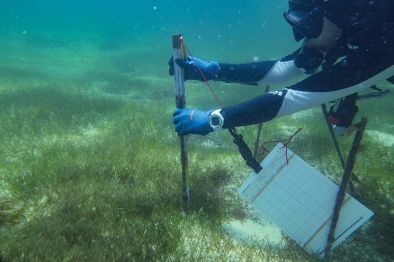This underwater photograph captures a scuba diver engaged in research or maintenance work beneath the ocean's surface. The scene features a horizontally aligned, rectangular composition. In the upper right corner, the diver, whose gender is indistinguishable, is visible from the arms up, wearing blue gloves and a navy and white diving suit. A white watch adorns their left wrist. The diver is either inserting or extracting a long, wooden-like stake with a white faceplate into the sandy, grass-mixed seabed. Attached to the stake is a rectangular, waterproof notepad or equipment gauge. Surrounding the diver, other long, black sticks or equipment pieces protrude from the ground, indicating an organized setup possibly related to the diver's task. The backdrop reveals bluish-green water filled with tiny bubbles, contributing to the serene, yet industrious underwater environment.